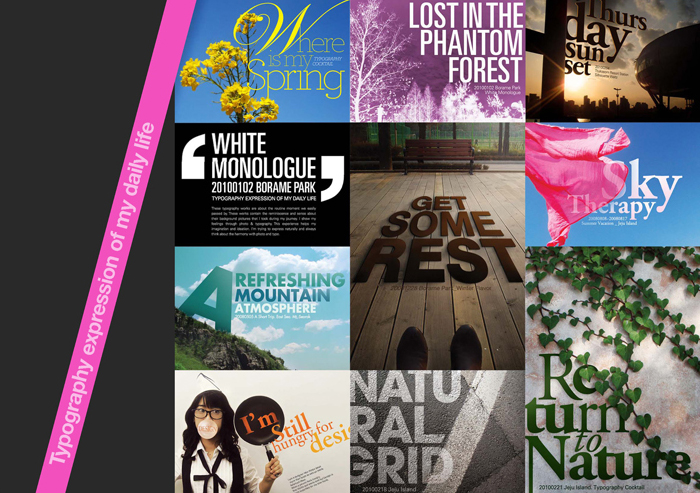This collage is a vibrant tapestry of various images, perhaps reflecting the creator's favorite readings or expressive moments captured through typography. Dominating the left edge is a pink line running from bottom to top, tilted slightly to the right, with white text that reads, "Typography Expression of My Daily Life." The images are organized in a grid format, each with distinct themes and text styles.

In the upper left corner, there is a square with the question "Where is My Spring?" Next to it is another square with a purple background that reads "Lost in the Phantom Forest." A sun setting behind a cross fills the next square down, captioned "Thursday's Sunset." Directly beneath it, against a black background, appears "White Monologue in Borham Park."

At the center of the collage is a larger square spanning two normal squares, with a wooden floor and a wooden bench in the background. Two pairs of feet are visible in front of it, accompanied by the text "Got Some Rest." On the right, an image with a blue background and a pink flag is captioned "Sky Therapy."

Below this, there’s a depiction of a mountain scene labeled "Refreshing Mountain Atmosphere." Next to it, an image features a girl in a white shirt with a black tie, wearing black glasses and a mask. She is holding up a frying pan and the text above reads "I'm Still Hungry for DESI."

Towards the bottom center, on a gray and white background, fragmented words spell "NATU," "RAL," and "GRID." In the bottom right corner, against a stone-colored background with descending leaves, sits the phrase "Return to Nature."

The dynamic collage serves as a visually rich narrative, melding diverse typography and imagery to convey distinct and personal sentiments, perhaps evoking a snapshot of the creator's daily life or current inspirations.